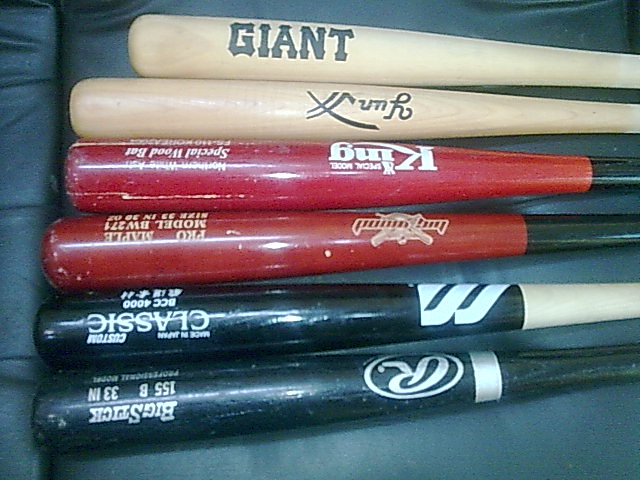The photograph showcases six baseball bats laid horizontally on a dark blue leather-like surface. Each bat is positioned with the barrel facing left and the handle out of sight. The top two bats are natural wood color and feature blue writing, with one of them prominently displaying "GIANT." Beneath these are two red bats, both adorned with black handles and white writing, including the brand name "KING" and "SPECIAL WOOD BAT." The black bat below these has a white handle and includes a logo and "PRO MAPLE MODEL BW271." Lastly, the bottom bat is completely black with inscriptions near the handle and reads "BIG STICK 155B, 33 INCHES" with a notable stylized "R" logo.